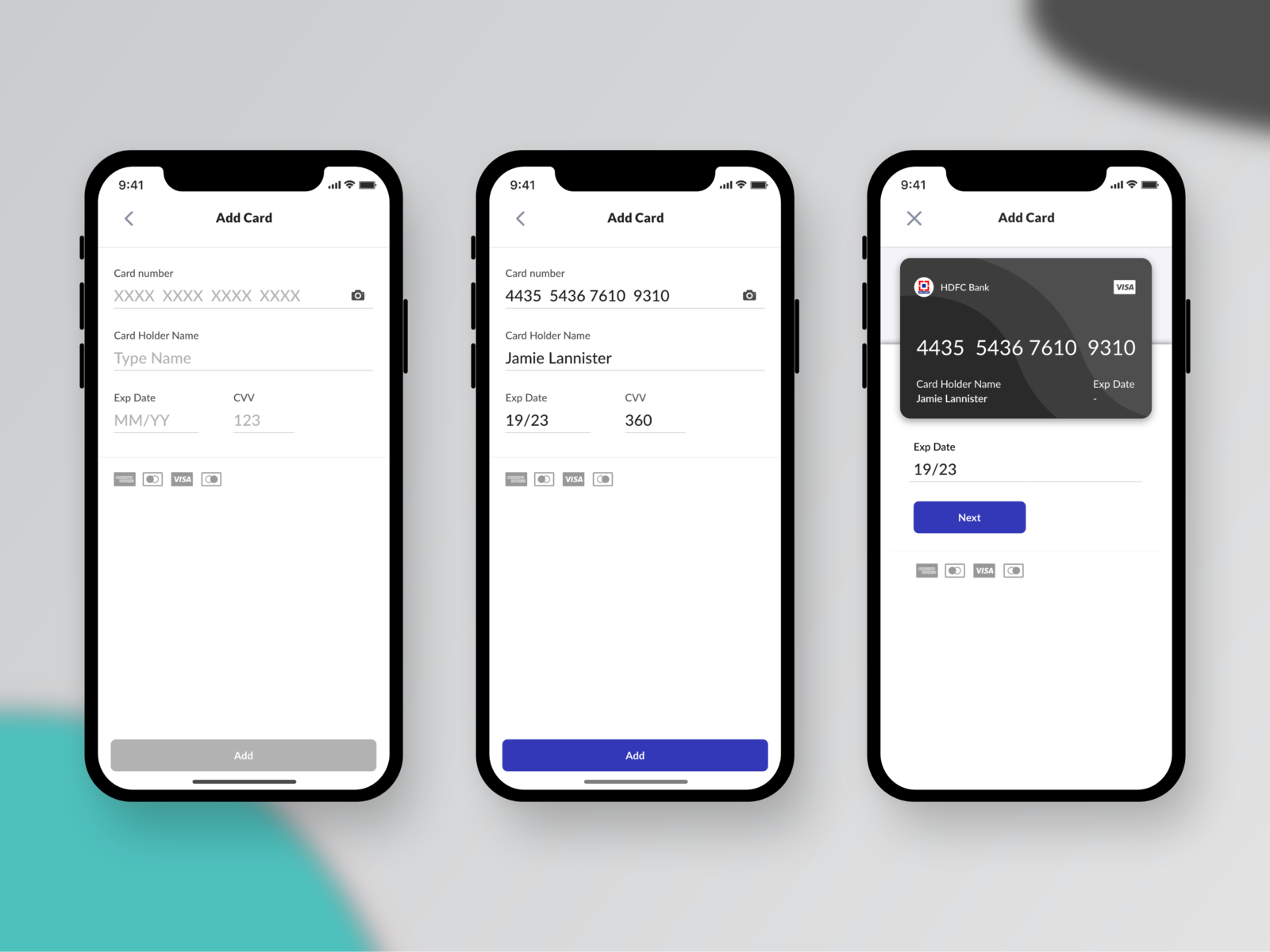The image displays a collage of three cell phone screens. The first screen, displayed on the left, shows a virtual credit card input form. At the top of the form, there's a header reading "Add Card." Below, the form fields include "Card Number" filled with 16 capitalized X’s, indicating placeholder text, and fields for "Cardholder Name," "Expiration Date," and "CVV," each with relevant placeholder text: "Type Name," "Month," "Year," and "CVV123" respectively. Small logos for credit card companies, including American Express, Visa, and MasterCard, are neatly arranged at the bottom of the screen.

The central screen features a partially filled-out form with the card number "4435 5436 7610 9310," the cardholder name "Jamie Lannister," and an expiration date marked as "1923."

The screen on the right showcases an image of a virtual credit card, prominently featuring the name "Jamie Lannister."